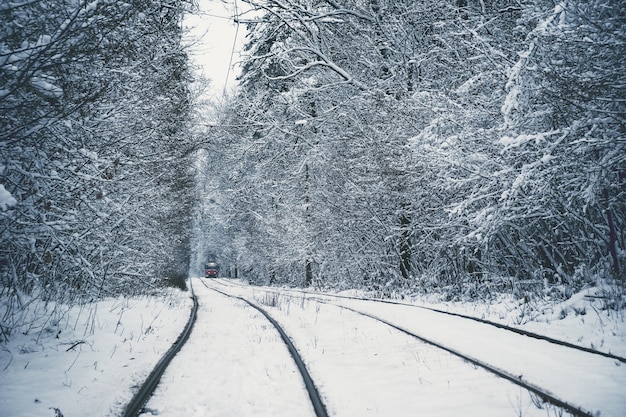This photo captures a cold, wintery railway scene dominated by snow and leafless trees. The ground is covered with a few inches of pristine white snow, forming a thin layer that blankets everything, including the two sets of train tracks running from the foreground to the distance. These tracks carve a path through a dense forest of trees, their branches bereft of leaves but heavily laden with snow. The sky, though visible, is a soft, featureless white, mirroring the snow-covered landscape below. In the distance, a reddish train with black windows or a black top is approaching on the right track, emphasizing the cold quietude of this outdoor scene. Additionally, an electrical wire runs above the tracks, suggesting that they support electric trains. The overall atmosphere suggests a serene but frigid winter day.